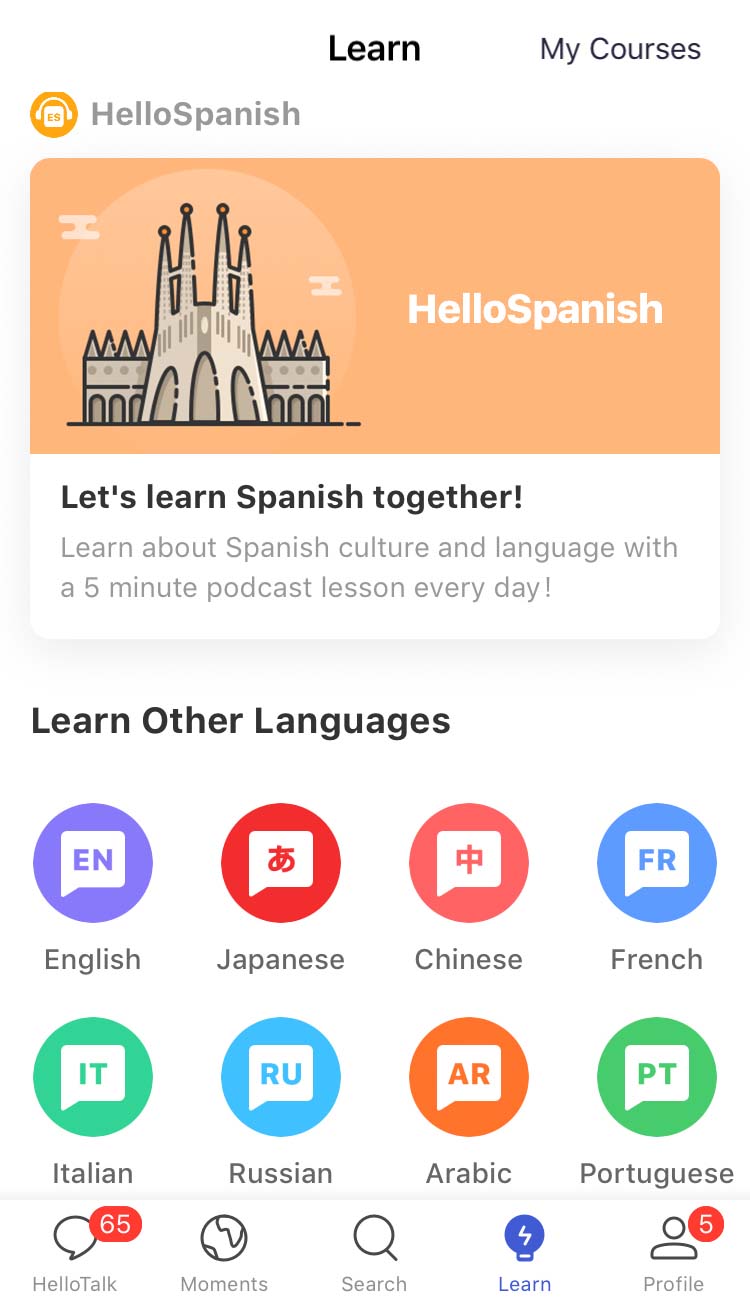**Hello Spanish Interface Overview**

The screenshot features the user interface of an app called "Hello Spanish," designed to facilitate learning Spanish. The background is shades of gray and white, giving the interface a clean and modern look.

- **Header Section:** 
  - At the top of the screen, there is an image of an orange castle with a distinctive design, including three arched windows and shorter towers on the sides, each topped with four pointed spires and small orange circles. 
  - To the right of the castle image, the text "Hello Spanish" is prominently displayed in white, written as a single word against an orange background. 
  - Above this, in gray, the same "Hello Spanish" text is repeated.

- **Navigation and Icons:**
  - To the left of the castle, there is a stylized "ES" box adorned with headphones, indicating an audio feature for Spanish learning.
  - Above this icon, the word "Learn" is displayed and bolded, suggesting it is the currently active section. 
  - To the right of "Learn," there is an option labeled "My Courses." 

- **Language Selection:**
  - Below the Hello Spanish header, there is a section labeled "Learn Other Languages." This includes buttons for several languages, each represented with a comment bubble icon:
      - English (EN)
      - Japanese (JA), with the Japanese symbol
      - Chinese (ZH)
      - French (FR)
      - Italian (IT)
      - Russian (RU)
      - Arabic (AR)
      - Portuguese (PT)

- **Additional Features:**
  - Beneath the language selection, there is another section labeled "Hello Talk," showing 65 notifications.
  - Adjacent to this are icons labeled "Moments," "Search," and "Learn" featuring a lightning bolt, indicating quick or instant learning sessions.
  - There is also a profile section with five notifications.
 
This well-organized interface combines linguistic tools and social features, encouraging a comprehensive and engaging experience for users who wish to learn and stay culturally connected with Spanish.